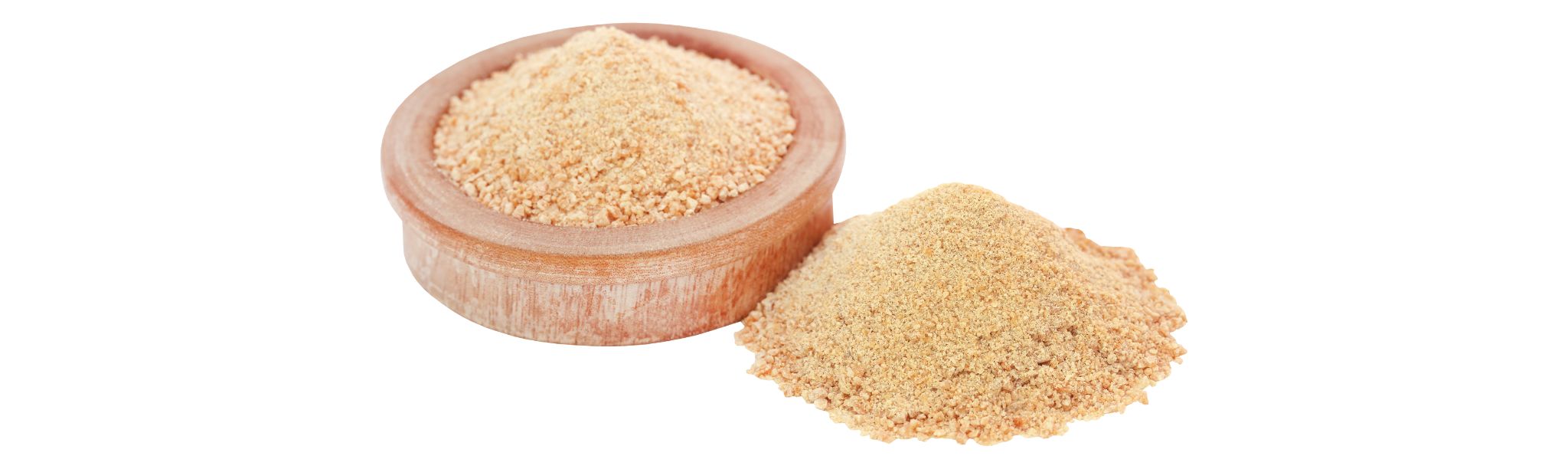In the photograph, a stark white background frames a scene with two distinct piles of powdery substance. To the left, a small, weathered clay bowl with a wide rim sits filled with light brown, finely milled powder, potentially indicative of flour or light brown sugar. The bowl, adorned with orange rust-like stains and striations, juxtaposes its rustic character with the purity of the setting. To the right of the bowl, on the pristine surface, is another mound of darker brown powder, resembling either processed grain or darker brown sugar. The variation in the brown hues suggests differing materials, spilling from the bowl to create a striking contrast against the white environment.